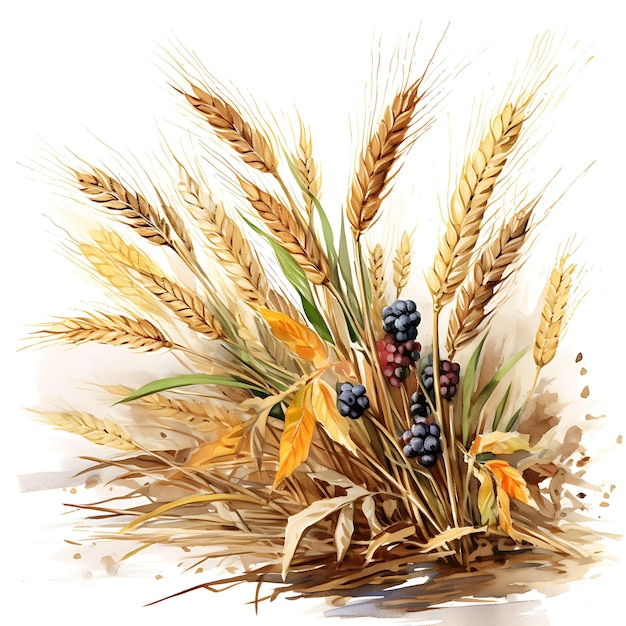This image appears to be a watercolor painting of assorted dried plants and flowers against a stark white background. The central focus is on wheat-like grasses with billowy, thread-like tops, colored a natural wheat hue. Interspersed among these are brown and orange leaves, as well as patches of green foliage on the left side. Distinctively, the middle section showcases clusters of berries, some a deep dark blue and others a lighter purple shade, resembling raspberries. Towards the bottom of the image, there are brown smears likely representing the ground. The painting lacks a visible signature, suggesting it might be cut off or not signed at all.